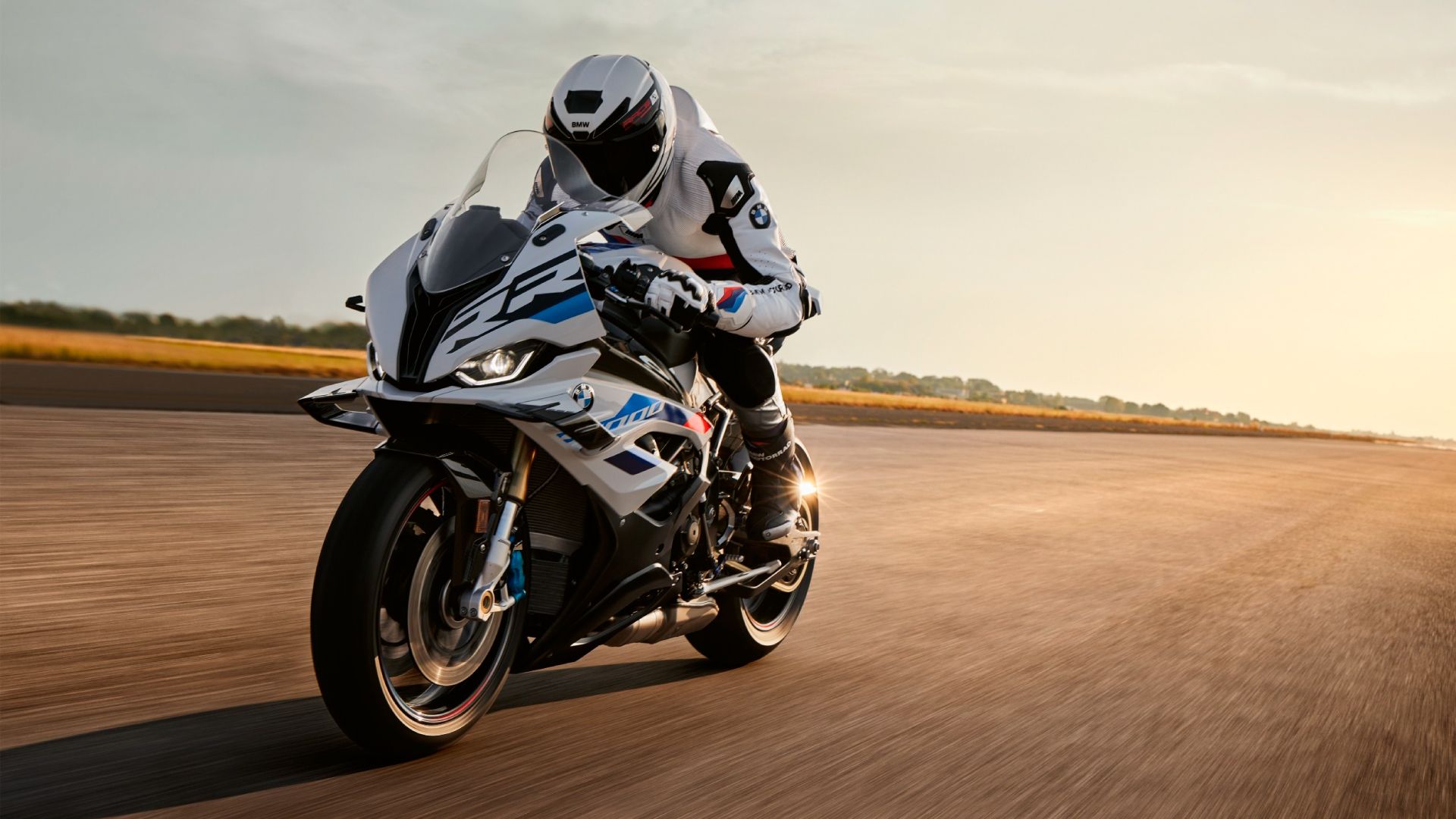In this outdoor daytime photograph, a man rides a white motorcycle accented with black, blue, and red, along a wide, brown, dirt road that stretches from left to right across the bottom half of the image. The motorcycle, positioned slightly left of center and moving towards the left, prominently displays a white “R” on a black streak on its front fairing beneath a small windshield, with blue and black detailing. The rider, dressed in a white and black motorcycle jacket with visible text on the left sleeve, black pants, white and black gloves, and black boots, leans forward in a tucked aerodynamic position. His helmet, matching his jacket in white and black, has a closed visor. To the left of the road, there is a field of pale yellow, possibly wheat, which extends into the distance, meeting a line of trees that spans the horizon. Above, a clear sky dominates the upper part of the image, providing a bright backdrop to the dynamic scene.